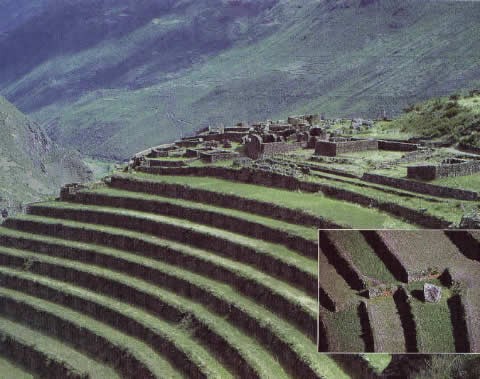This grainy composite photograph captures the awe-inspiring ruins of Machu Picchu set against a mountain backdrop. The main image, dominating most of the frame, showcases the terraced hill crowned by ancient ruins. A shallow-sloping, predominantly green mountain with gray shadows occupies the upper third of the photograph. In the foreground, lush terraces lined with dark gray stones lead up to the ruins. The terrace sides are meticulously constructed, each terrace slightly offset from the next. At the summit of these verdant steps lies the remnants of what appears to have been an elaborate settlement. The structures, built from gray stone, include curved walls that align with the terraces and an array of right-angled buildings indicative of Incan architecture.

The inset image in the bottom right corner offers a close-up of a specific terrace section, revealing detailed stonework and a prominent large gray stone sitting on one of the steps. This smaller photograph highlights a particular area of interest, which is suggested to possibly be an entrance, perhaps to an underground tunnel, adding an element of intriguing mystery to the historic site.